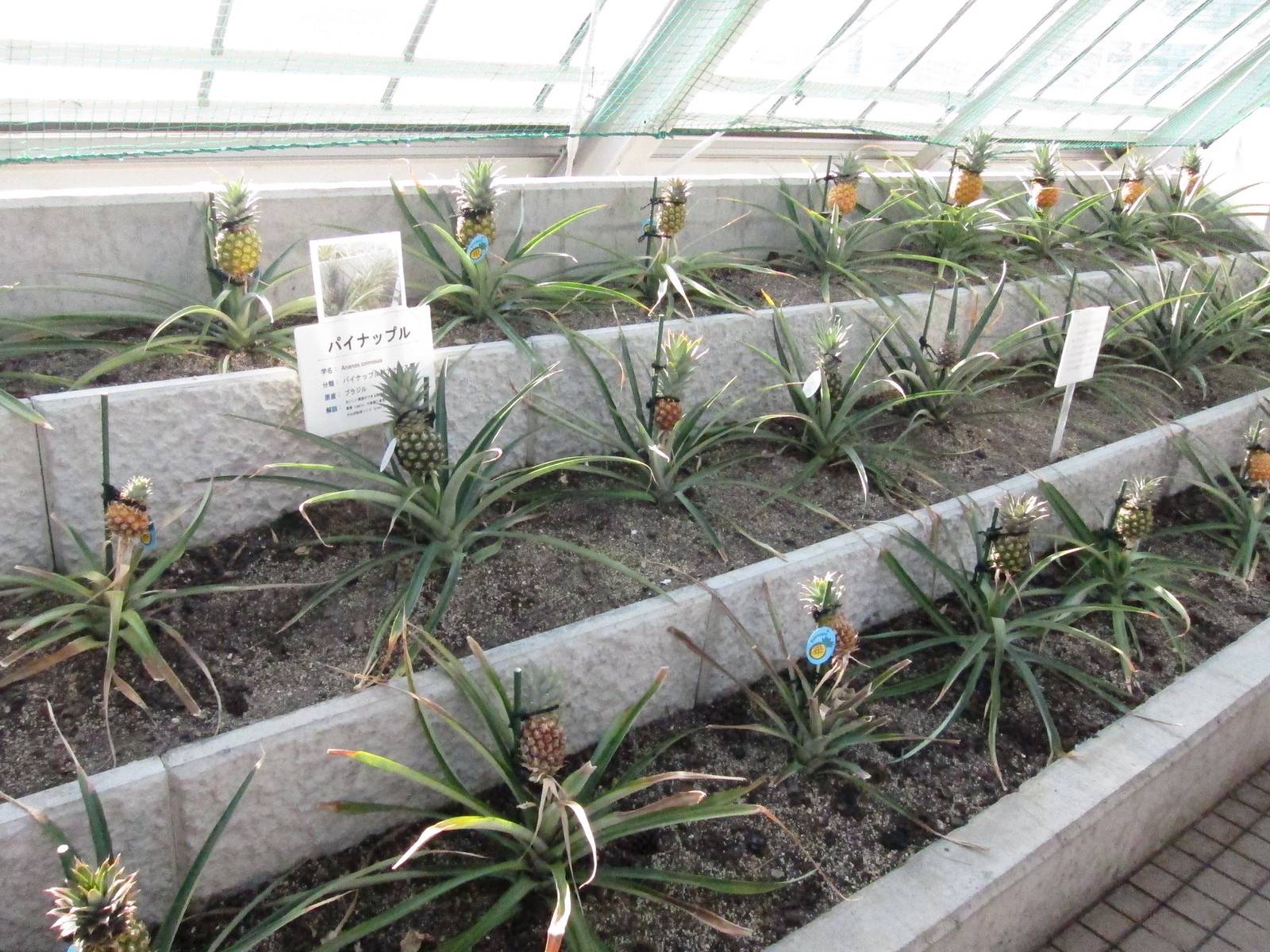The photograph captures the interior of a commercial greenhouse in Japan, distinguished by signs in Japanese katakana that label the varieties of pineapples being cultivated. The greenhouse is organized into three tiers, each with rows of plants growing tiny pineapples. The plants, which have long, thin leaves, are spaced about a foot apart in uniform rows, and are planted within grey concrete planters. Above, a series of slanted glass windows allow sunlight to filter through, enhancing the cultivation environment. Additionally, a tiled walkway is visible in the bottom right corner of the image, suggesting accessibility within the greenhouse. The arrangement and detailing of this greenhouse indicate a meticulous and systematic approach to growing different species of pineapples.